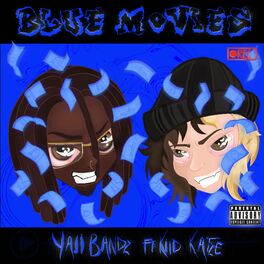The album cover, rendered in a low-quality, small image, features a chibi, anime-style illustration of the two musicians presumably behind the album. Dominated by a blue color palette, the cover has a central blue rectangle bordered by black on the top and bottom. At the top, the title "Blue Movies" is visible in black text with a blue outline. The bottom text reads "Yaji Bands featuring Kid Catzy," although it is somewhat difficult to discern clearly due to the low image quality and hand-drawn, JPEG-distorted lettering.

In the center of the cover, the chibi portraits show two artists. On the left is a black individual with dreadlocks, glasses, and a nose ring. On the right is a white individual wearing a black beanie, with two-toned, dark brown and blonde hair, sharp teeth, red-tinged eyes, and a vampire-like appearance. Their eye features give an impression of them being under some influence, suggested by their reddened eyes.

Additionally, the cover includes a Parental Advisory sticker on the bottom right corner, and a recording notification is drawn at the top. Surrounding the portraits, there appears to be a visual element resembling money or pieces of paper falling around their heads.